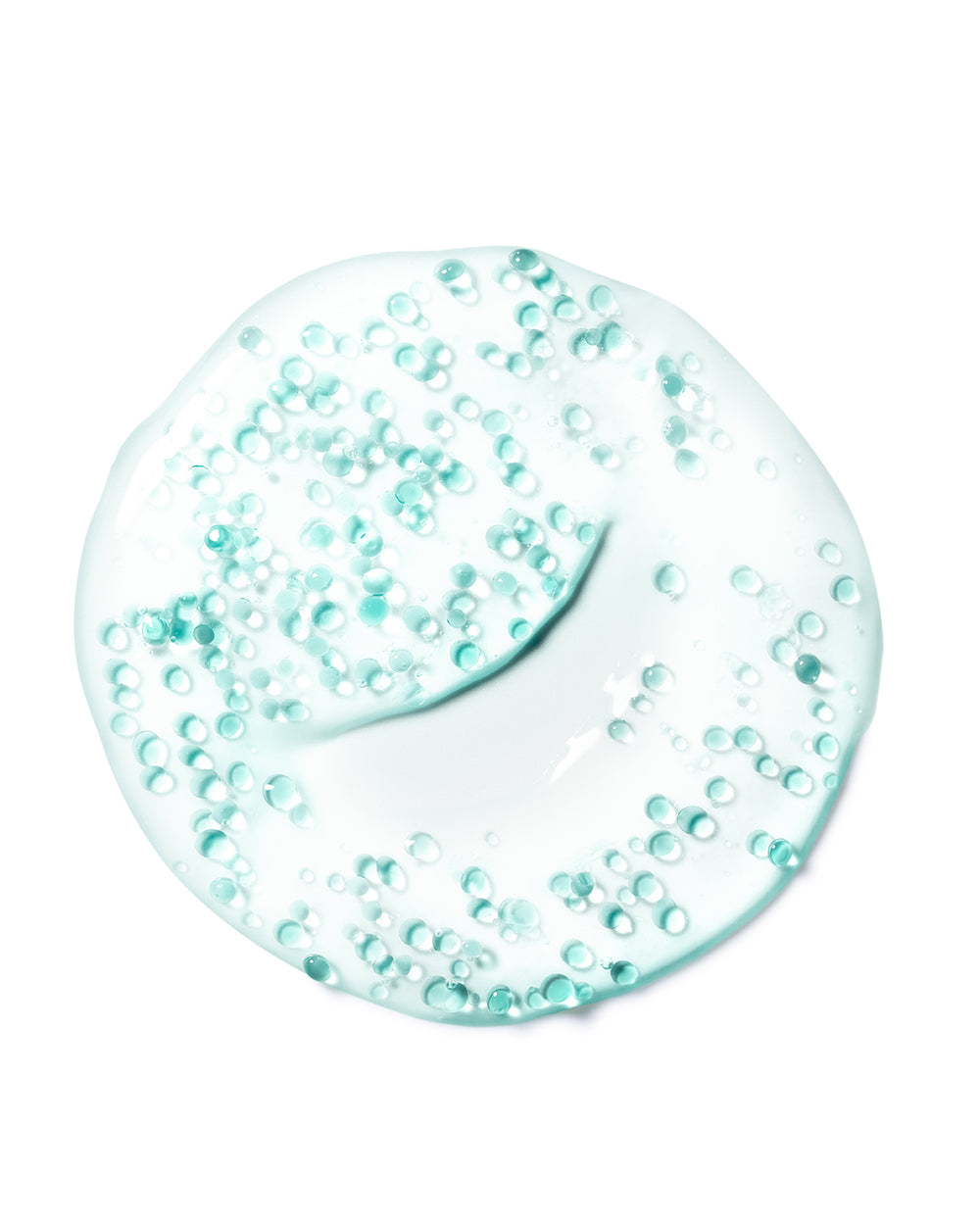The image depicts a slightly lopsided, circular-shaped, pale bluish-green viscous blob set against a white background. This blob is interspersed with numerous tiny bubble-like droplets, predominantly focused on the upper left and center regions. Notably, there is a noticeable gap towards the middle right where fewer bubbles are present. A darker curved line running through the blob adds contrast, creating an impression reminiscent of a mouth. These droplets vary from clear to different shades of green, including pale mint and emerald, giving the overall appearance a subtly green hue. The precise nature of the image remains ambiguous, leaving room for interpretation as either a microscopic view of a liquid or a scientific or chemical substance.